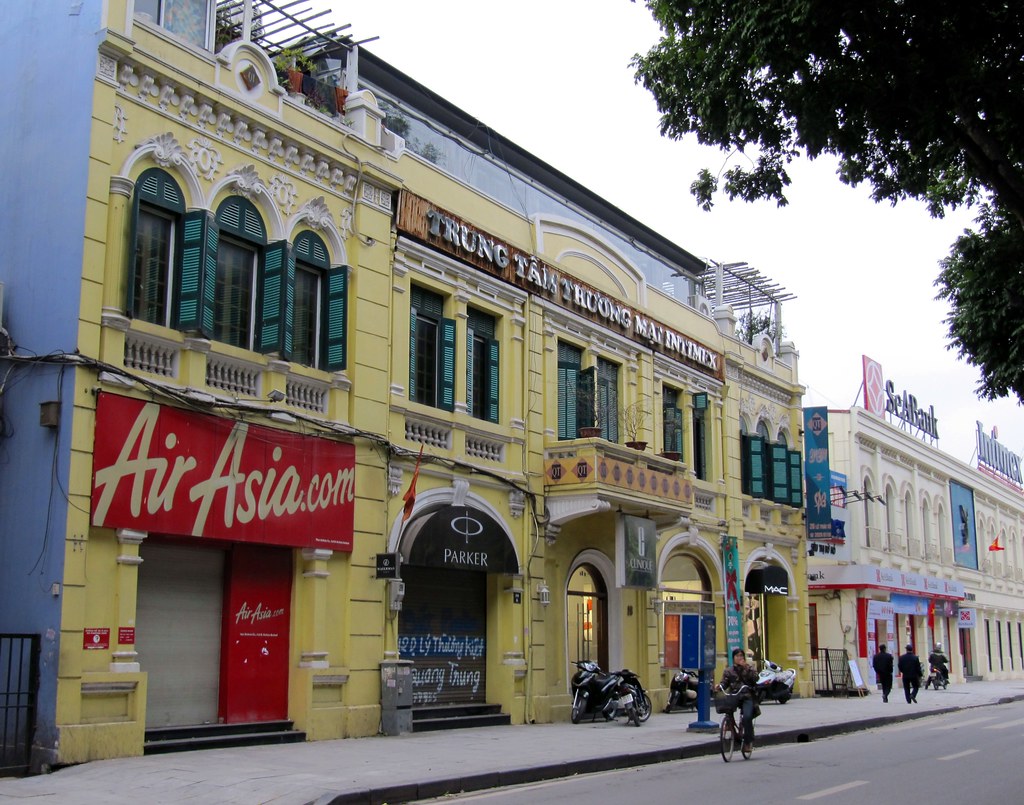This vibrant street scene, likely set in Vietnam, showcases a commercial urban block with two distinct buildings side by side. The first building, painted a vivid yellow, features ornate architectural designs and a variety of retail stores at street level, including AirAsia.com, Parker, Clinique, and MAC. Above these shops, the upper level displays numerous windows and a sign with Vietnamese text, possibly reading "Tran Thanh Thang Mai Intimix." Adjacent to this is a white building, which appears to house a bank on its ground floor. This bustling street is animated by pedestrians, a bicyclist, and several mopeds and motorcycles parked or navigating the area. In the background, green-framed windows and a rooftop adorned with vases and plants can be seen, adding a touch of greenery to the urban landscape. A tree's branches and leaves extend into the upper right corner of the image, completing the lively street scene bustling with daily activity.